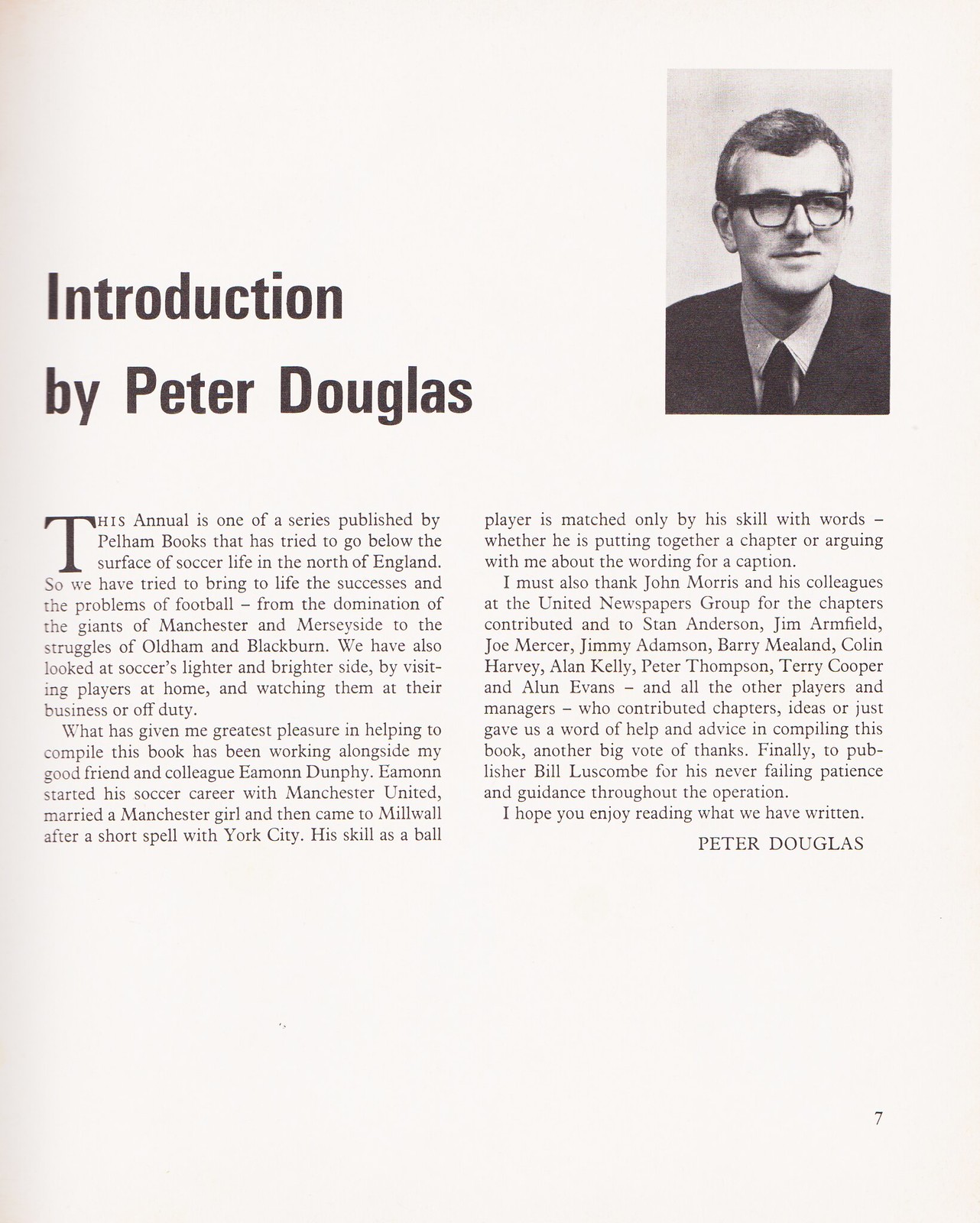This image depicts a page from an introduction, most likely from a book or a magazine, appearing on page seven. The page has a light white background with a significant amount of black text. The top right-hand corner features a black-and-white photograph of a man with salt-and-pepper hair and thick black-rimmed glasses. He is dressed in a black suit, with a white collared shirt and a dark tie, and wears a serious expression while looking slightly to the right.

On the left side of the page, in dark font, the text reads "Introduction by Peter Douglas." Below this heading are two side-by-side paragraphs. The first paragraph starts with, "This annual is one of a series published by Pelham Books that has tried to go below the surface of soccer life in the North of England." It continues to discuss the aims of the publication, which include bringing to life the successes and struggles of football teams from prominent clubs like Manchester and Merseyside to smaller clubs such as Oldham and Blackburn. 

The text also mentions exploring the lighter aspects of soccer by visiting players in their homes and observing their off-field activities. The second paragraph includes acknowledgments and thanks to colleagues, players, and those who assisted the author in compiling the book, ending with Peter Douglas expressing his hope that readers will enjoy what he has written.